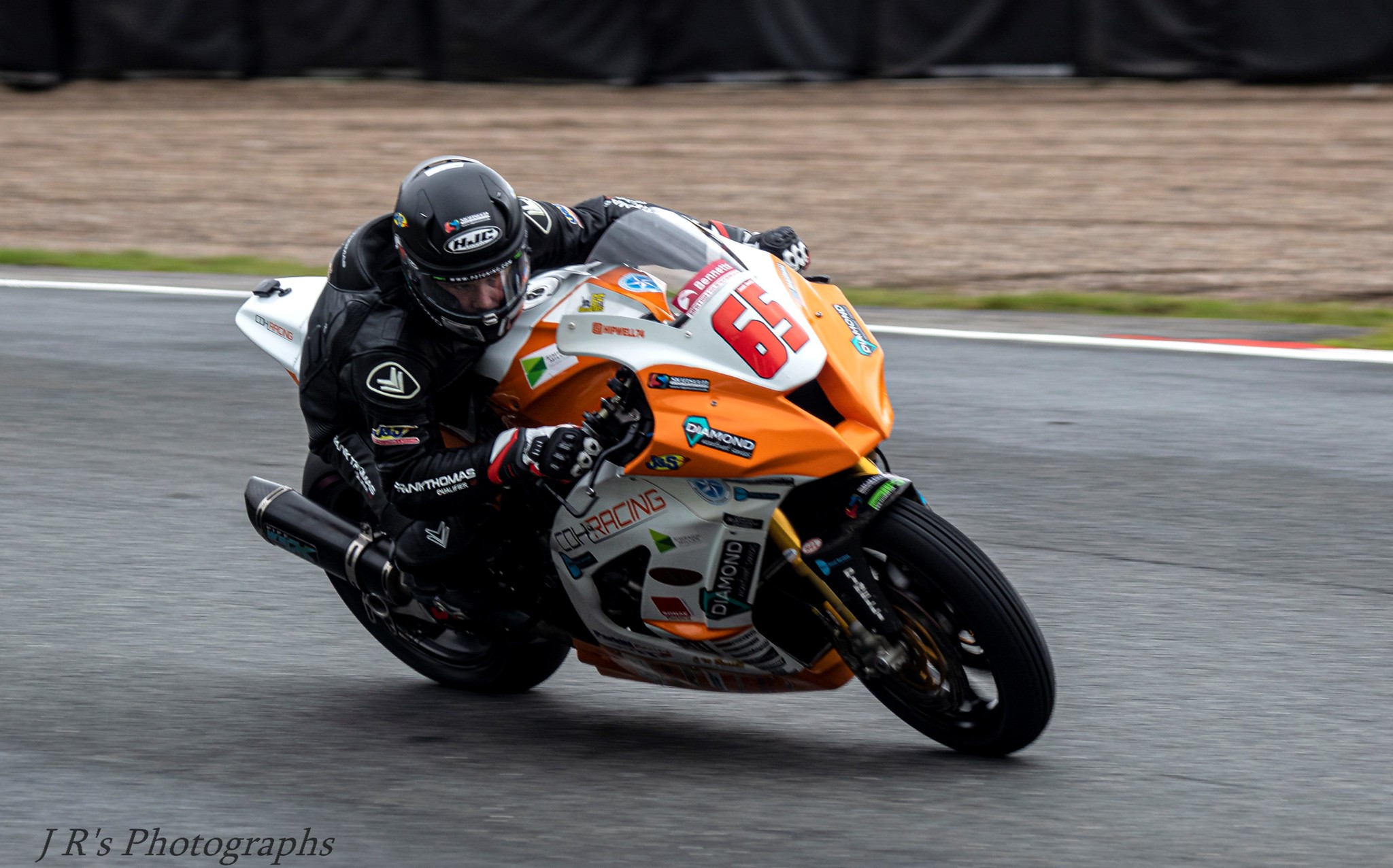The action-packed photograph captures a determined motorcyclist in mid-race, skillfully leaning into a curve on a dark gray asphalt track. The rider, clad in a black racing suit adorned with sponsor logos, matches his black gloves and shiny black helmet. His intense focus is evident as he controls the white and orange sport bike marked with the number 65 in red on its front. The motorcycle's sleek design includes orange trim and black wheels, emphasizing its racing prowess. The background features a distant, flat brown field and a darker area resembling a wall, contrasting with the track's white border. At the bottom left corner, the image is watermarked with "JR's Photographs" in black italicized text, marking the image's professional capture.